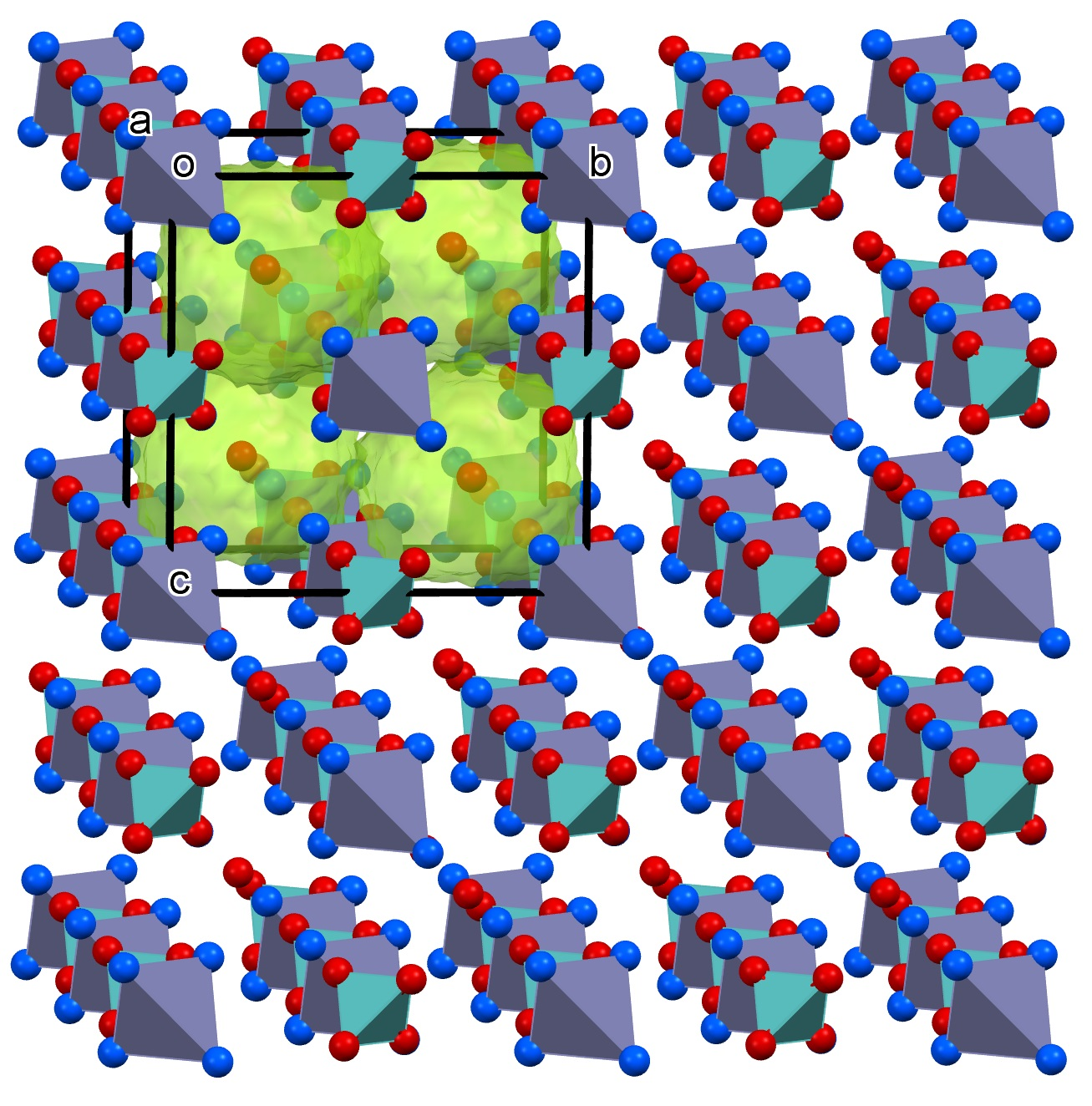The image is a scientific diagram illustrating a 5 by 5 grid of molecular structures. Each structure within the grid is composed of two primary overlapping triangles: a dark blue triangle with its shallow point at the bottom left and a lighter blue triangle with its shallow point on the right. The corners of these triangles are marked with blue spheres. Positioned behind these is a yellow triangle with its corners attached to red spheres, and this entire pattern is repeated twice, creating a layered effect. Some of these structures feature an additional red sphere on the yellow triangle. 

The top left structure is labeled "A" and "O" in black text with a white outline. The third structure from the left is labeled "B," and the third structure down on the left is labeled "C," using the same text style. In the top left quadrant, there is a translucent green box outlined with a thick black line, containing more of these molecular structures visible behind it. The background of the entire diagram is white, enhancing the visibility of the grid and the elements within it.